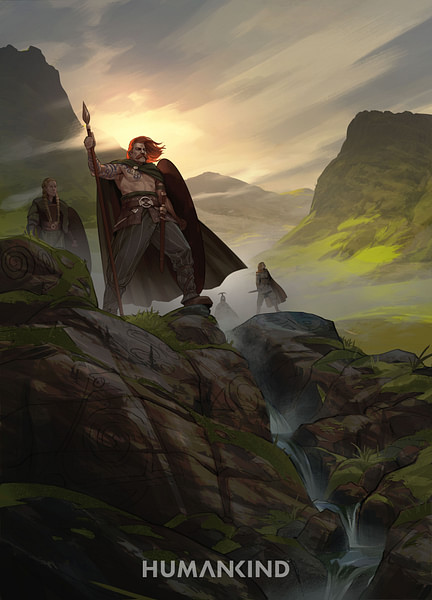This piece of artwork, which could be for a fantasy comic book, animation, movie, or video game concept, depicts a dramatic and detailed scene set in a fantasy landscape. In the foreground, a large man with flowing red hair and a mustache stands resolutely on a moss-covered rock formation by a small stream. He is clad in striped black pants, a brown leather belt, and a long green cape, but is shirtless. The man wields a spear with its point resting on the ground and a large, body-length wooden shield in his left arm. Behind him stands a woman with braided blonde hair, also equipped with a shield. In the background, slightly obscured by fog, are two additional figures. The setting includes bright green grassy cliffs and a towering, green-colored rock cliffside to the right, with the sun piercing through the clouds, giving the scene a muted, atmospheric light. At the bottom of the image, the word "HUMANKIND" is prominently displayed in all caps, with a distinctive combined "K" and "N" in the font.